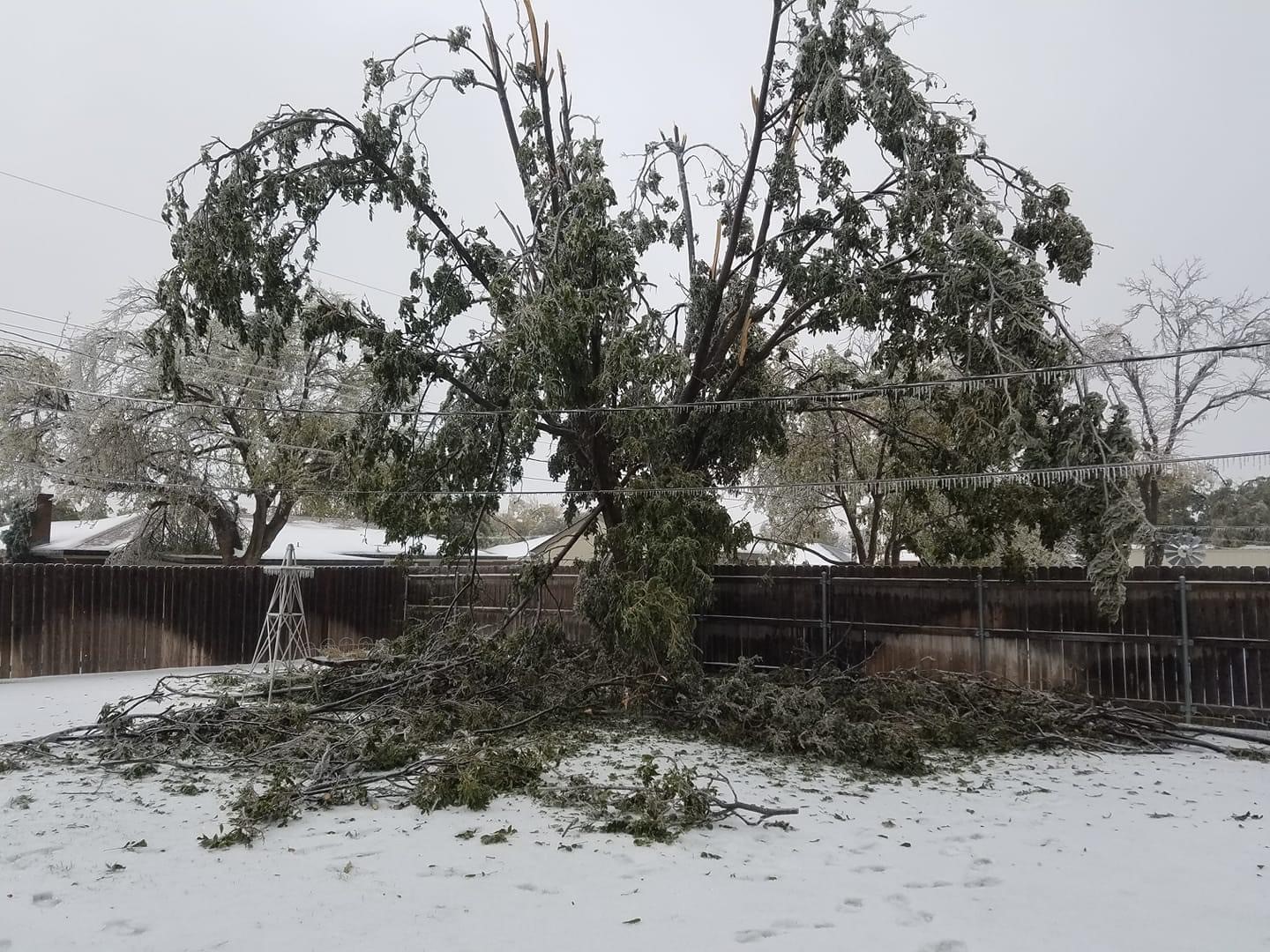A color photograph captures a winter scene in a fenced yard dominated by a large, heavily ice-laden tree at its center. The tree, likely felled by a recent storm, shows significant damage: many of its limbs have broken off from the main trunk and now lie scattered across the snow-covered ground. Some branches remain green but droop under the weight of the ice. The brown wooden fence stands amidst the debris of leaves, branches, and sticks, partially obscured by the fallen limbs. Overhead, power lines stretch across the yard, hanging heavy with icicles. In the background, other trees, similarly laden with ice but still standing, add to the dreary, gray wintry atmosphere. The scene is one of stark contrast between the vitality of the remaining greenery and the overall desolation wrought by the ice storm.